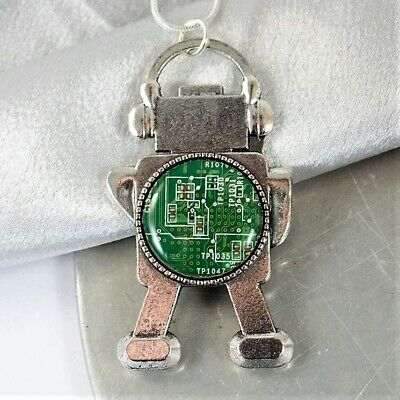The image is a detailed close-up photograph taken indoors, featuring a robot-shaped keychain set on a surface that combines a white cloth on its upper half and a scratched, grayish metallic surface on the lower half, possibly a table. The robot, primarily made of steel, sterling silver, or platinum, exhibits a distinct color transition from brown and light copper at the bottom to silver at the top. It has a rectangular head with ear-like protrusions and a loop for attaching the keychain. The body is square at the base and rounded at the top, integrating a large green circular element on its chest that resembles a circuit board, bordered by silver dots. This creates the impression of peering inside a complex technological device. The robot’s design is enhanced with two small arms, appearing folded behind its back, and two legs with a wide stance, giving the impression of a sturdy, well-balanced structure. Additionally, elements on the robot's head evoke headphones, while a serial number is inscribed on its body, emphasizing its intricate, artful construction.